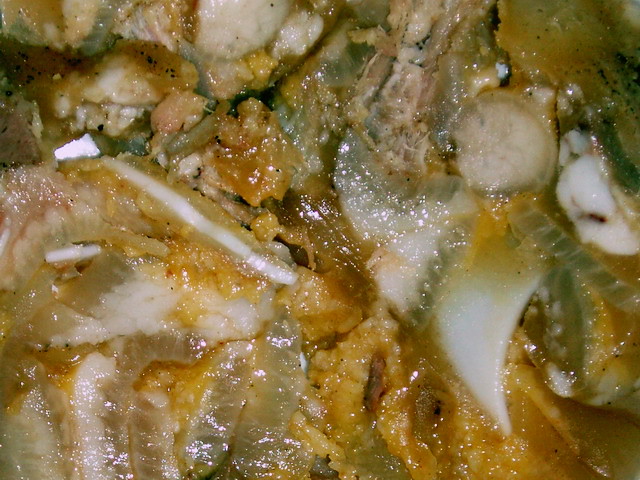The image is a close-up, detailed and rather unappetizing view of a slimy, gooey, and moist substance that is difficult to identify. It features a mix of colors, including white, yellow, green, and orange, with a jelly-like, segmented appearance. The white areas resemble tendons or flat noodles, while the yellow and greenish sections look squishy and gummy-like. There are also some tiny black dots scattered throughout the orange parts. It appears to be covered in a sauce, possibly an orange type, giving it an even more unappealing, wet look. The zoomed-in perspective makes it hard to determine if it is food, animal parts, or something else entirely.